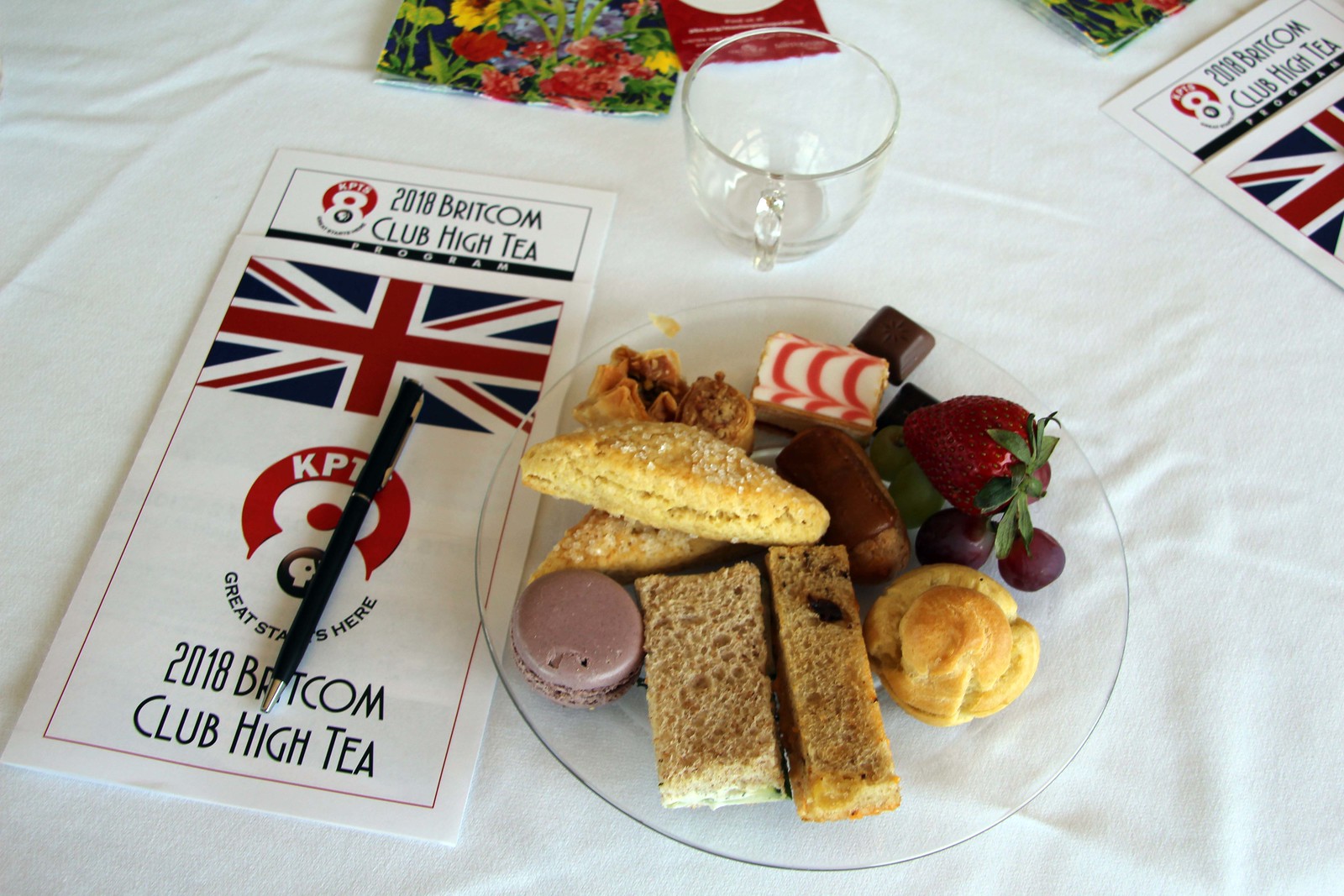On a table with a white tablecloth, a clear glass plate in the center carries an array of treats including two pieces of bread, a couple of pastries (one topped with sprinkles), a round purple pie, and a slice of pie with white and red layers. A strawberry, a couple of cherries, a square of chocolate, and what appears to be a chocolate macaron, a curry puff, and a mini doughnut are also on the plate. To the right of the plate, there is an empty clear glass cup with its handle pointing downward. To the left of the plate, a menu prominently displays the title "2018 Britcom Club High Tea," accompanied by an image of a British flag. The menu also includes the text “KPT” with a black pin underlined by the number 8, bears the slogan "greatest stats here," and is repeated on another identical menu in the upper right corner of the scene. Beside the cup and towards the center back, there are two additional cards, one decorated with flowers and the other featuring a red bottom. The overall display suggests a British high tea setting, with other pamphlets spread across the table, indicating multiple participants at this event. The dominant colors in the image are red, white, blue, and black.